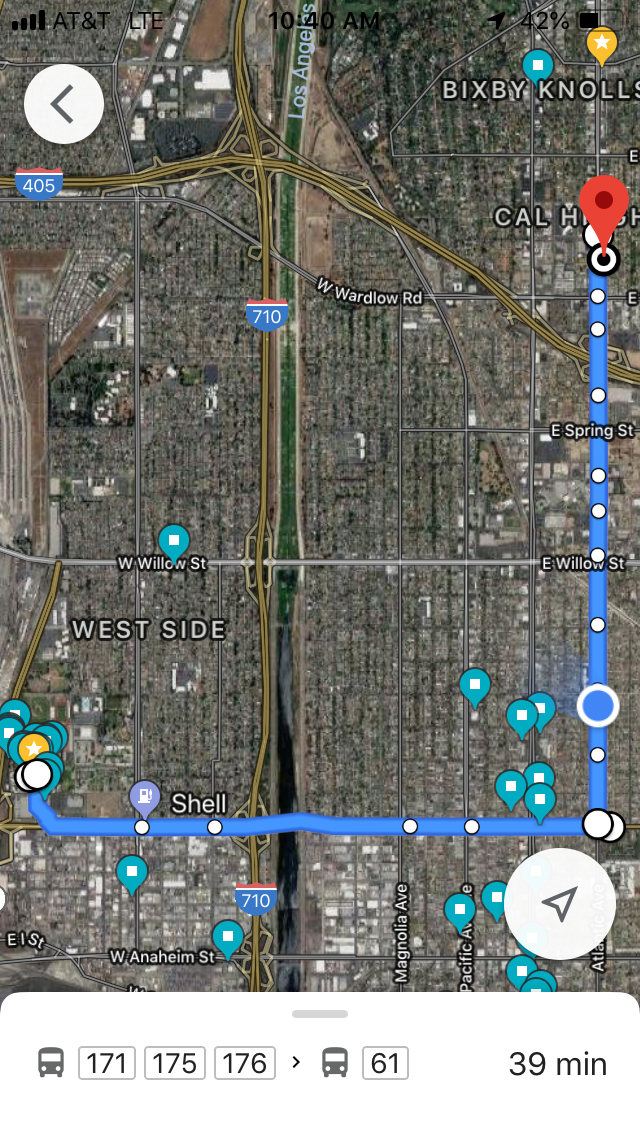The image displays the screen of a mapping application on a smartphone, showcasing a detailed map of a section in Los Angeles. The map prominently features a network of streets and two intersecting highways. The north-south running highway is labeled 710, while the east-west highway is designated as 405. Key streets visible on the map include West Wardlow Road, West Willow Street, Magnolia Avenue, and West Anaheim Street. Additionally, the map provides a bird’s-eye view of buildings scattered below, adding a layer of urban texture to the scene. The map's comprehensive layout highlights the intricate connectivity of the city's roads and highways.